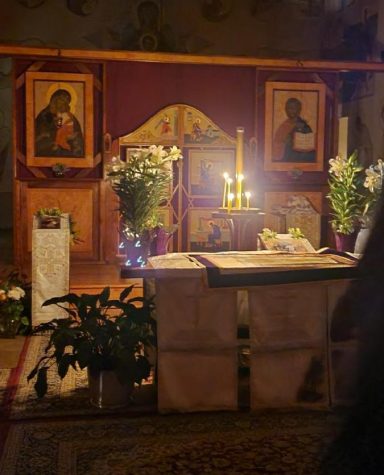The image depicts a somber funeral altar situated in a dark, muted room that appears to be a place of worship. The focal point is a large table covered in rich textiles and linens that drape to the floor. This table is adorned with numerous candles, casting a soft glow that illuminates the otherwise dim space. Flanking the table are pots of blooming peace lilies and Easter lilies, adding a touch of life to the solemn scene. The floor is covered with geometric oriental rugs that overlap slightly at the center.

In the background, a maroon wall is decorated with intricate tapestries and four religious paintings. The top two paintings clearly depict saints with halos, framed in natural wood. A natural wood shelf runs above these paintings, adding an element of rustic charm. Amidst these decorations, an arched doorway is visible, centrally positioned between the paintings, suggesting an entryway into a deeper sanctum. The room's dark ambiance, accentuated by the burgundy and deep hues of the textiles, creates a sacred and introspective atmosphere.